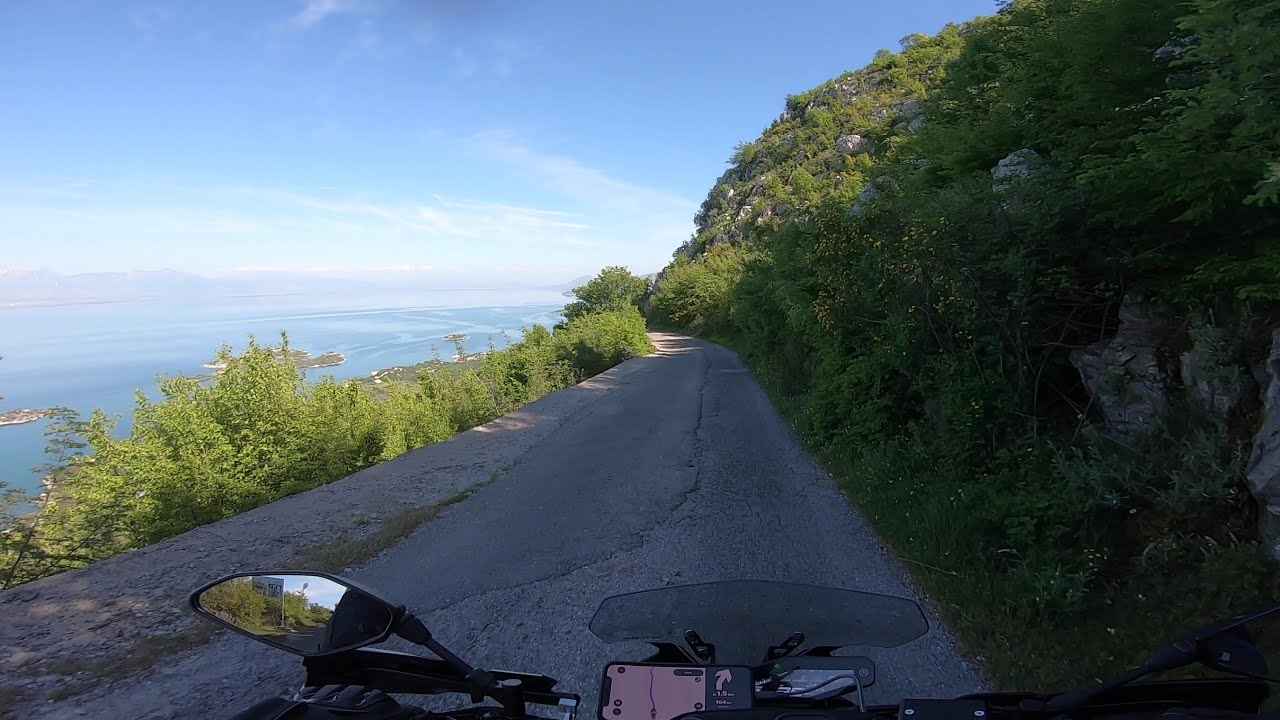The image portrays a captivating view from a biker’s perspective, displaying a scenic and adventurous journey. The biker’s gloved left hand is visible near the bike’s handlebar, with the left side mirror prominently in view and a small part of the right side mirror peeking into the frame. Mounted just below the front windshield of the motorcycle, an iPhone displaying a GPS app has a white arrow indicating a right turn. The narrow, paved road stretches ahead with a rough, rocky, and bushy hillside on the right side. To the left, the road dramatically drops off into a cliff, exposing a large body of shimmering blue water, presumably an ocean or a lake, with some small islands in the distance. Green vegetation flanks both sides of the road, accompanied by a few scattered trees. Above, the sky is a striking blue, dotted with just a few light clouds, adding to the breathtaking tranquility of this countryside scene.